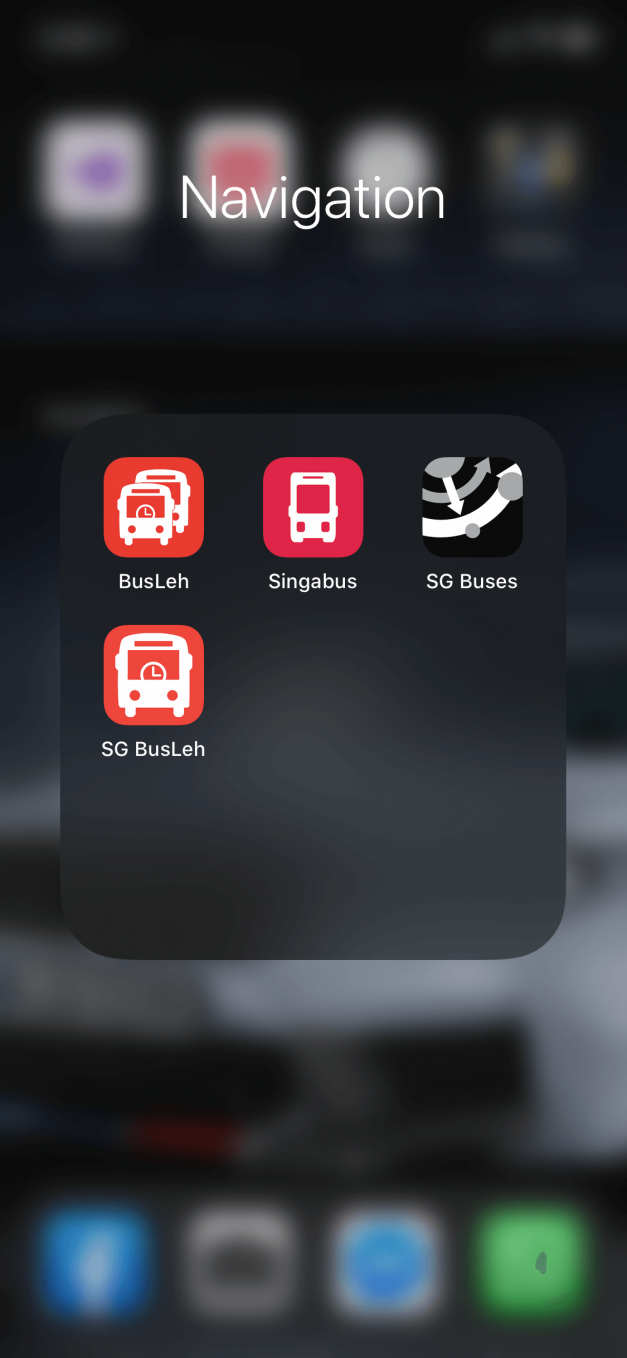The image contains a blurry background and features a series of icons and objects. At the top, there are several boxes, each with an icon in its center. One of the icons appears to be the YouTube logo, while the others remain unidentified. At the bottom, there are four icons aligned in a row. The far-left icon is the Facebook logo, with two more central icons that are indiscernible, and a green icon on the far right. Above these icons is a gray object, also out of focus.

Additionally, there's a dark gray pop-up menu with navigation options prominently displayed. The pop-up menu contains four square icons. The top-left icon is in a red square and depicts a bus labeled "Bus L-E-H." To its right is another red square with a bus labeled "Singer Bus." Further to the right is a third icon with gray stripes, labeled "SG Buses."